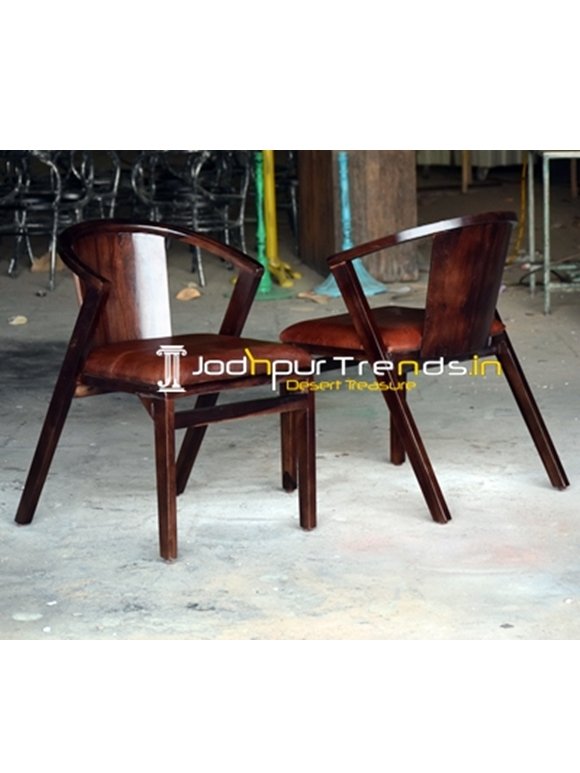This slightly landscape-mode color photograph showcases two modern and elegant wooden chairs with dark mahogany or cherry wood finishes and leather cushions on the seat. The chairs, featuring unique diagonal back legs, are placed on a white floor that appears somewhat dirty, hinting at a workshop setting. One chair is facing forward while the other is positioned backward, offering a view of its compact backing. Behind these chairs, metallic seating can be seen, reinforcing the warehouse atmosphere. Prominently displayed in the middle of the image is a modern-styled logo reading "Juwampur Trenzin Desert Treasure," with the text in alternating white and yellow hues.